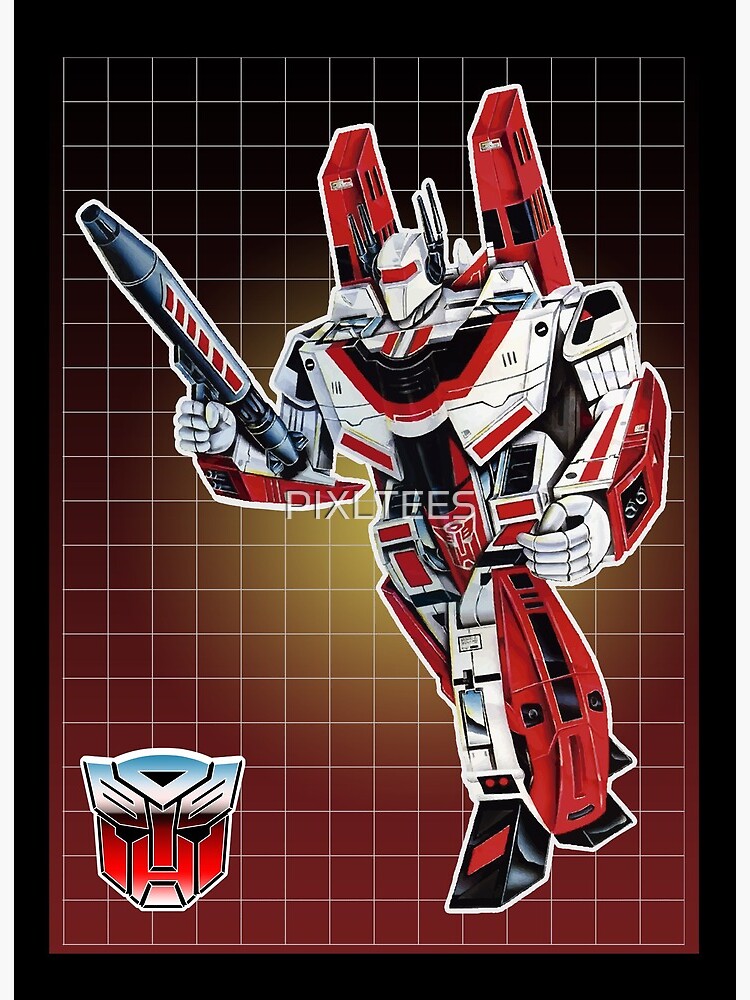This is a horizontally oriented digital drawing featuring the G1 version of Jetfire, a Transformer, prominently displayed on the right. Jetfire is depicted with intricate mechanical and humanoid features, including angular arms, legs, and a helmeted head. His color scheme features a dominant white with vibrant red accents on his legs, arms, and backpack, black detailing, and red eyes. Holding a long, narrow black gun in his right hand, which is on the left side of the image, Jetfire appears to be moving forward. The background showcases a gradient grid pattern transitioning from black at the top to yellow in the center and red at the bottom. In the lower left corner, the Transformer logo—a red face with black eyes and a white top—is visible. The entire image is bordered in black, and a semi-transparent watermark reading "PIXLTES" spans the center.